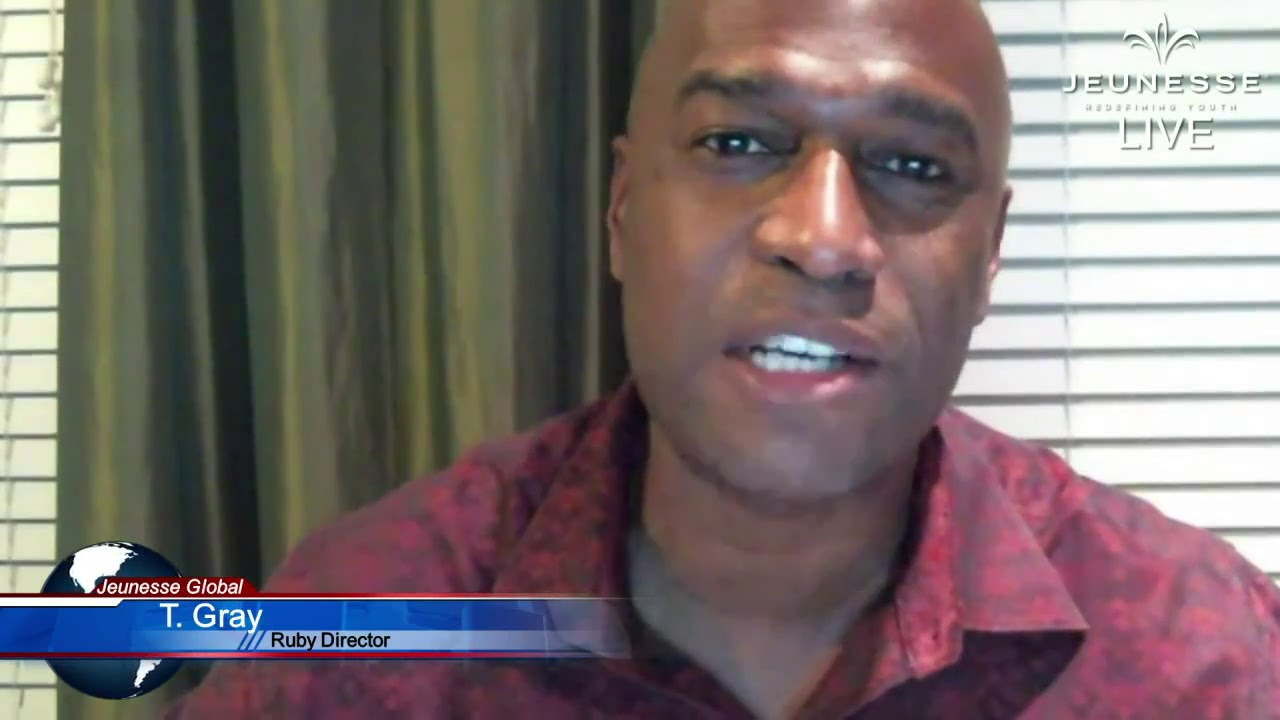The image portrays a close-up still shot of a dark-skinned man, identified as T. Gray, speaking during what appears to be a televised interview. T. Gray is slightly off-center to the right and is wearing a striking red collared shirt, partially open at the neck, revealing his white teeth as he speaks. His dark brown eyes are slightly visible, and he is bald or balding. The backdrop includes white horizontal blinds and green curtains positioned behind his right shoulder, offering a simple and professional setting, possibly an office.

In the top right corner, the text "Jeunesse Live" is displayed in white against a contrasting background, and a small logo is evident above the text. The bottom left corner features a blue banner with red borders, containing the text "Jeunesse Global" in white. Below this, the name "T. Gray" is prominently displayed, indicating his title as "Ruby Director" in black text. A subtle image of the Earth is visible behind the banner, adding to the global theme of the presentation.